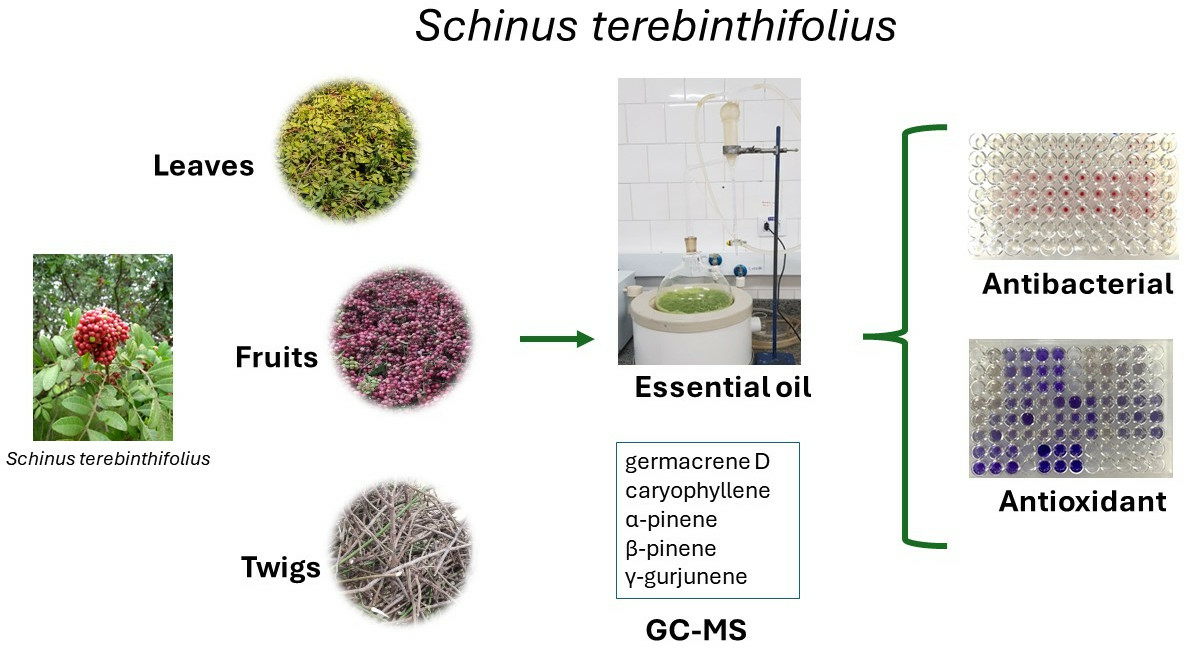The diagram illustrates various components and properties of the plant Schneebus terebinthus. On the left side, there is an image of the plant labeled "Schneebus terebinthus," followed by detailed photos of its leaves, fruits, and twigs, each accompanied by corresponding text. An arrow points to a container labeled "essential oil," depicting the extraction process. Below this container, a box lists chemical compounds including germicrine D, caropheline apn, bpn, and y-gergine, with "GC-MS" (Gas Chromatography-Mass Spectrometry) indicated underneath. On the right side, two small grids are presented; the top grid is red and labeled "antibacterial," while the bottom grid is blue and labeled "antioxidant."